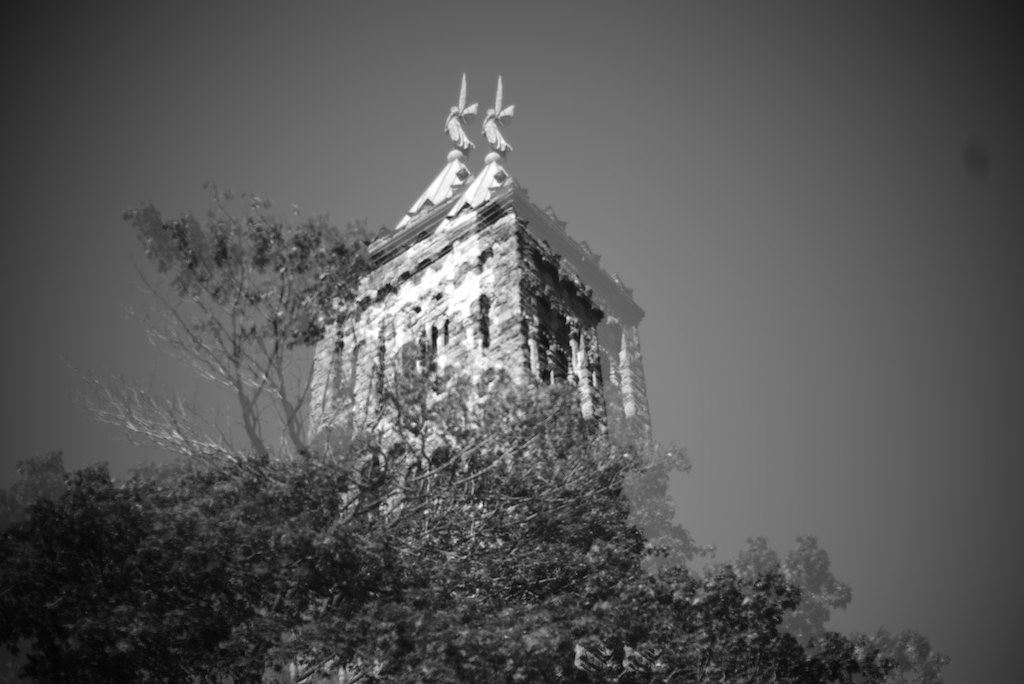This black and white photograph captures a striking scene that appears to be designed for viewing with 3D glasses, as it exhibits a double vision effect. At the center of the image stands a brick structure resembling a castle tower, topped with a pyramid-shaped roof. Crowning the peak of the roof is a metallic angel statue. The base of the structure, possibly a mausoleum or an art piece, is surrounded by trees and dense vegetation, indicating a serene yet somber setting, like a graveyard. The photo is taken from ground level, looking up towards the angel statue, emphasizing the grandeur and majesty of the scene.